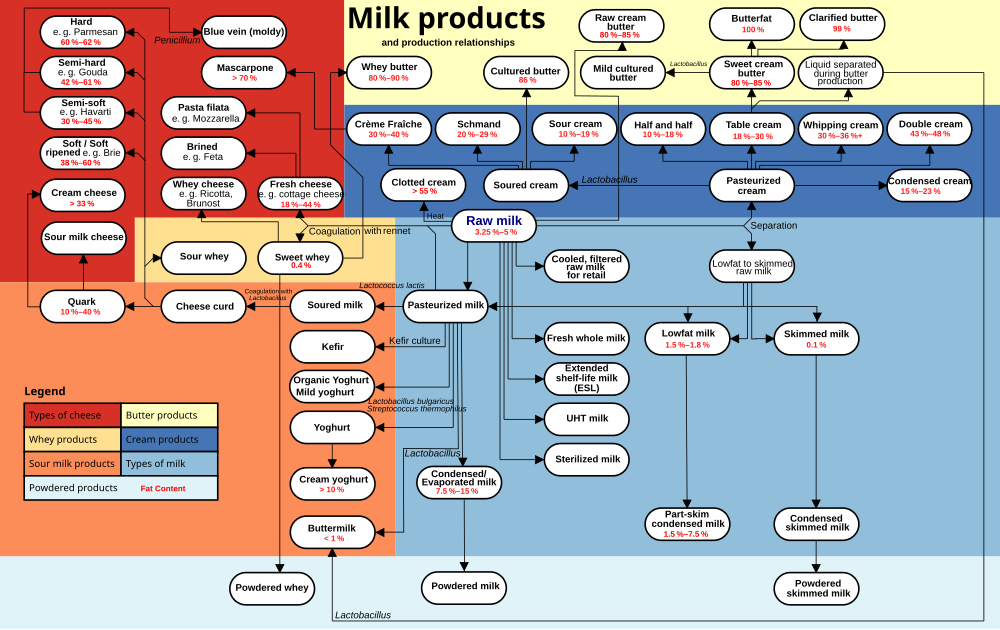This is a highly detailed and color-coded graph, presented in the image, that illustrates various milk products and their production relationships.

- **Cheeses (Red)**: The left side of the graph lists different types of cheese, starting from hard Parmesan to soft varieties and including options like semi-hard Gouda, semi-soft Havarti, soft Brie, cream cheese, sour milk cheese, blue-veined mold cheese, mascarpone, pasta filata, mozzarella, brined feta, whey cheese, ricotta, brown cheese (brunoise), fresh cream, and cottage cheese.
- **Whey Products (Tan)**: This section details sour whey and sweet whey.
- **Sour Milk Products (Coral)**: It includes quark, cheese curd, soured milk, kefir, organic yogurt, mild yogurt, yogurt, cream yogurt, and buttermilk.
- **Powdered Products (Light Blue)**: Listed here are powdered whey, powdered milk, and powdered skim milk.
- **Butter Products (Cream)**: At the top of the graph, it categorizes whey butter, cultured butter, raw cream butter, mild cultured butter, butterfat, clarified butter, sweet cream butter, and the liquid separated during butter production.
- **Cream Products (Dark Blue)**: This segment covers creme fraiche, schmand, clotted cream, soured cream, sour cream, half-and-half, table cream, pasteurized cream, whipping cream, double cream, and condensed cream.
- **Types of Milk (Light and Medium Blue)**: These include raw milk, cooled filtered raw milk for retail, low to skimmed raw milk, pasteurized milk, whole fresh milk, extended shelf milk, UHT milk, sterilized milk, low-fat milk, skimmed milk, condensed evaporated milk, part-skim condensed milk, and condensed skim milk.

**Legend**: The graph features a legend on the left, with colors indicating different types of products:
- **Red**: Types of cheese
- **Coral**: Whey products
- **Orange**: Sour milk products
- **Light Blue**: Powdered products with fat content
- **Cream**: Butter products
- **Dark Blue**: Cream products
- **Medium Blue**: Types of milk

This graph serves as a comprehensive visual representation of the relationships between various milk derivatives and product categories.